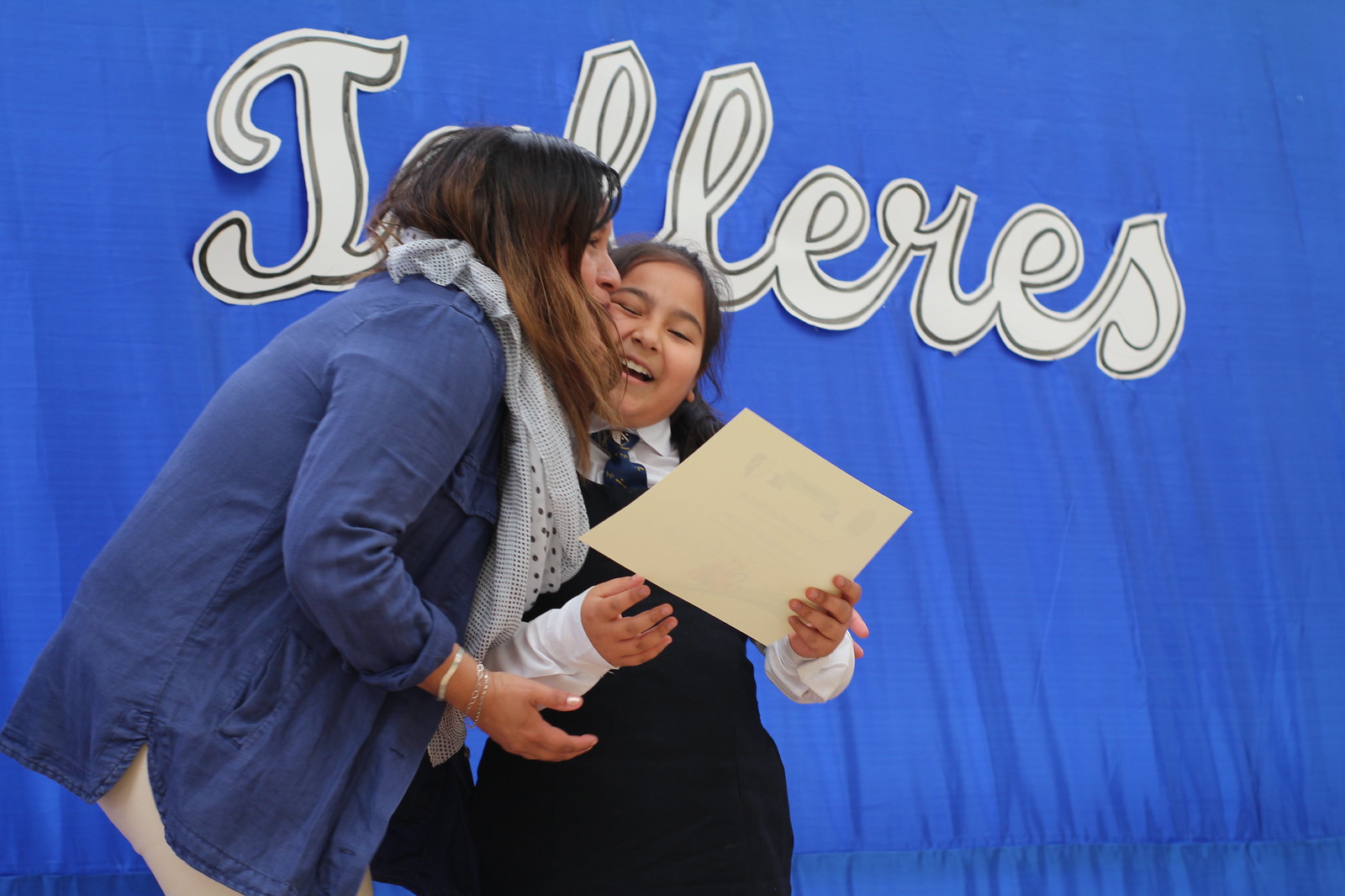This is a photo of an older woman and a young girl standing together in front of a vibrant blue curtain adorned with white cursive letters, partially obscured by their heads. The letters spell something that appears to contain the sequence "J-L-L-E-R-E-S." The woman on the left has straight brown hair and is wearing a blue button-down shirt paired with a large, decorative white scarf. She is affectionately kissing the cheek of the smiling girl, who looks around seven or eight years old. The girl has long brown hair tied up and is dressed in a navy blue school uniform—a jumper over a white button-down shirt with a blue tie. She holds a piece of paper in her hand, possibly a certificate or award. The interaction portrays a moment of pride and joy as the woman celebrates the girl's accomplishment.